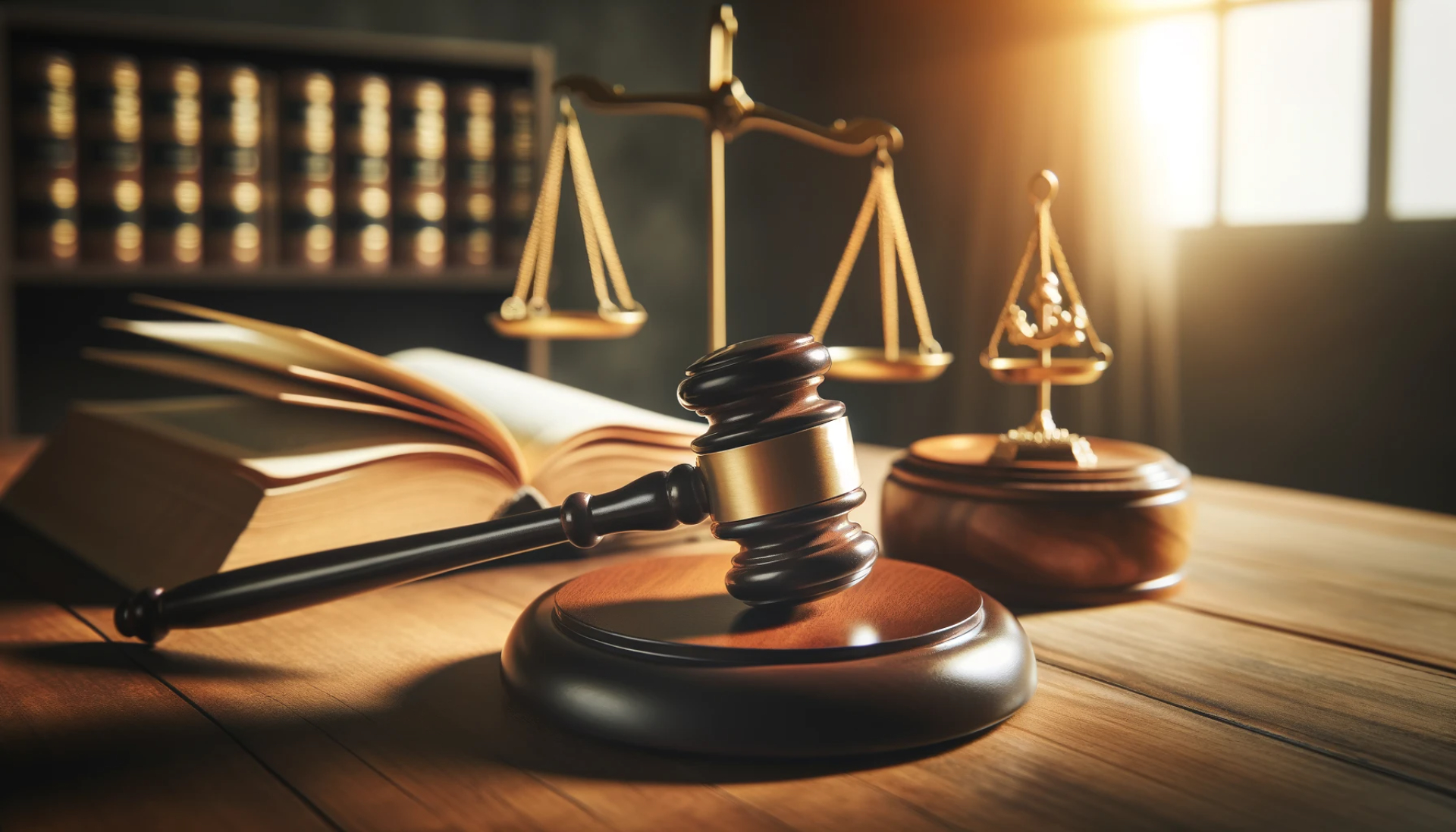This image captures what appears to be a judge's desk, characterized by a cohesive brown color scheme. Central to the composition is a wooden gavel resting on a striking base. Next to the gavel, an open book with thick pages catches the eye, though the text is not discernible. Adding to the scene's judicial ambiance, a gold scale, perched on what appears to be a wooden base, slightly leans towards the right. Another prominent item on the desk is a round container with a golden handle, possibly an anchor, suggesting a maritime or legal motif. The desk is set against a backdrop of a fully stocked bookshelf, indicative of law books or encyclopedias, alongside a window with open blinds that allow sunlight to pour into the room, casting a warm glow on the scene. The overall setting, enriched with wooden and golden elements, conveys the authoritative atmosphere of a judge's office.